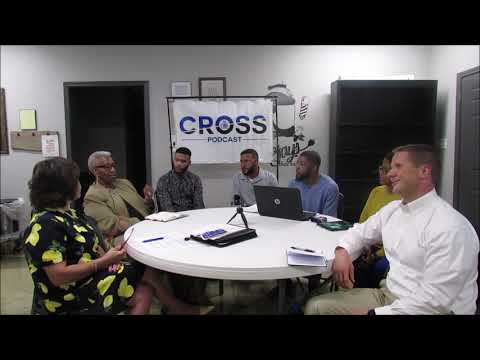The image depicts a professional meeting set in an office environment characterized by minimalist decor. Seven individuals, dressed in business casual attire, are seated around a white round table. The group comprises four males and three females of diverse ethnic backgrounds, including three black individuals, two white individuals, and one person of each ethnicity. One of the attendees, a man in a blue long-sleeved shirt, is using a laptop, while others have notebooks and pens, suggesting note-taking or discussion. 

The focal point of the background is a white banner adorned with blue text that reads "CROSS Podcast," indicating that the meeting might revolve around podcasting activities. The banner is affixed between two vertical poles and features a black border. Complementing the banner, the room has white walls with various decorative elements, including painted drawings and framed pictures in white and brown frames. Additionally, an empty black bookshelf stands against the right side of the wall, and there's an open doorway to the right of the banner that adds depth to the scene. The room's color palette is a mix of white, black, gray, and brown, with a tannish floor, underscoring the minimalist design. At the center of the table, there appears to be podcasting equipment set up on stilts, highlighting the purpose of the meeting.